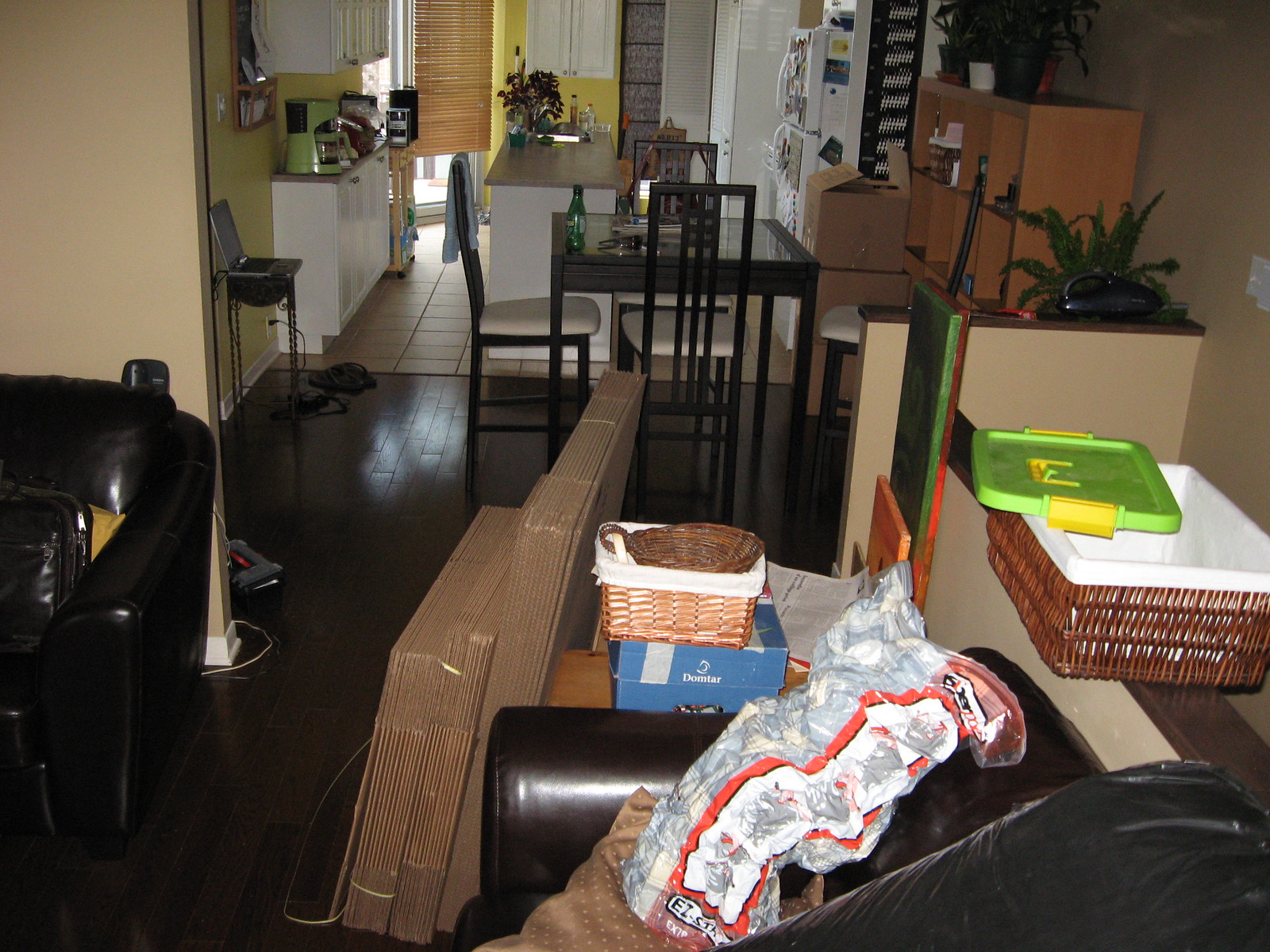This color photograph captures the interior of a house or apartment in the midst of a move. In the foreground, part of a brown leather couch is visible, with its right arm supporting a plastic or cloth bag and a brown pillow. Nearby, a large stack of unopened moving boxes, still strapped and plastic-wrapped, leans vertically against a side table. The side table itself holds a blue box, likely filled with trash bags, and a cloth-lined wicker basket with another smaller round basket nested inside it.

To the left, there is another black leather-look couch juxtaposed against a beige wall. Dark hardwood floors stretch across the room, adding a rich contrast to the lighter furnishings. Behind the right-side couch, a large wicker basket with a cloth lining sits alongside a lime green and yellow lid from a plastic storage bin. There is a shelf or bookcase behind this, holding a plant and divided cubicles, filled with assembled cardboard moving boxes.

Set in the middle of the room is a square dining table accompanied by four modern ladder-back chairs featuring white upholstered seats. The table displays a green glass bottle and some plates, indicative of a meal or gathering. This area flows into a galley-style kitchen, characterized by tile flooring and sunny yellow walls. The kitchen's left side is lined with white base and wall cabinets, accented by a lime green appliance on the counter and an open laptop on a small side table.

A yellow wall extends to the back of the kitchen, where sliding glass doors covered by bamboo roller shades allow light to filter in. The right side of the kitchen hosts a white refrigerator adorned with various magnets. The overall scene suggests a lively and dynamic household in the process of settling into a new space.